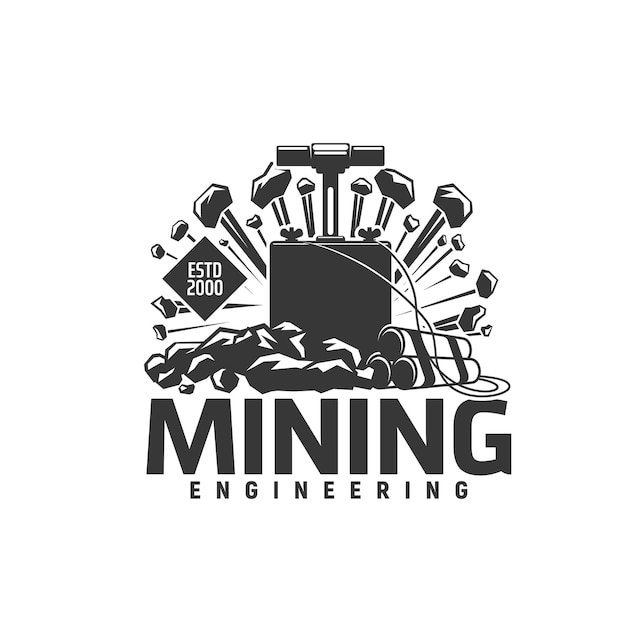The image is an advertisement or company logo for "Mining Engineering," displayed in bold, uppercase text at the bottom. The detailed, black-and-white design above the text features a dynamic mining scene centered around a traditional dynamite detonator. The detonator box, fully black with a prominent press-down handle, connects via wires to three bound sticks of dynamite on the right side. This explosive setup is depicted in action, with rocks and debris visibly bursting outward from the detonation point, illustrating the force of the explosion. To the left of the detonator box, a small black diamond shape with white text reads "ESTD 2000," indicating the establishment year of the company. This logo cleverly combines elements of mining tools and dynamism, strikingly visualizing the essence of mining engineering.